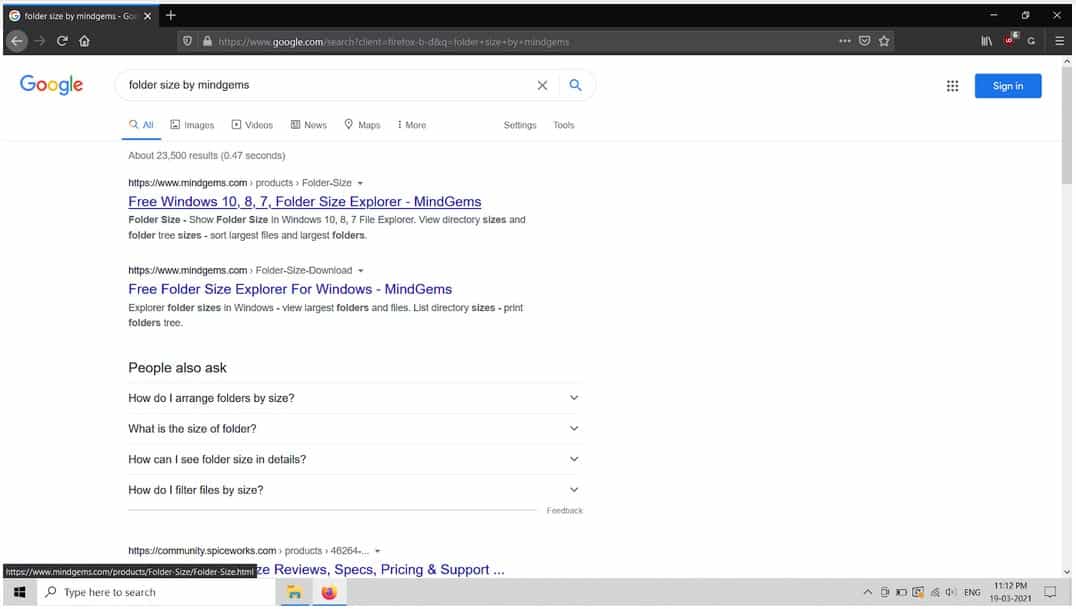The image captures a screenshot of a web browser displaying a Google search results page on a computer. 

At the top of the page, the Google logo is prominently displayed, adjacent to the search bar which contains the query "folder size by Mind Gyms." Below the search bar, the search results are visible. The first two search results are similar:
1. "Free Windows 10.8.7 Folder Size Explorer - Mind Gyms."
2. "Free Folder Size Explorer for Windows - Mind Gyms."

Further down the page, there is a "People also ask" section, listing four questions:
1. "How do I arrange folders by size?"
2. "What is the size of a folder?"
3. "How can I see folder size in details?"
4. "How do I filter files by size?"

In the top right-hand corner, there is a blue "Sign in" button. The entire web page has a clean, all-white background, with black text for easy readability.